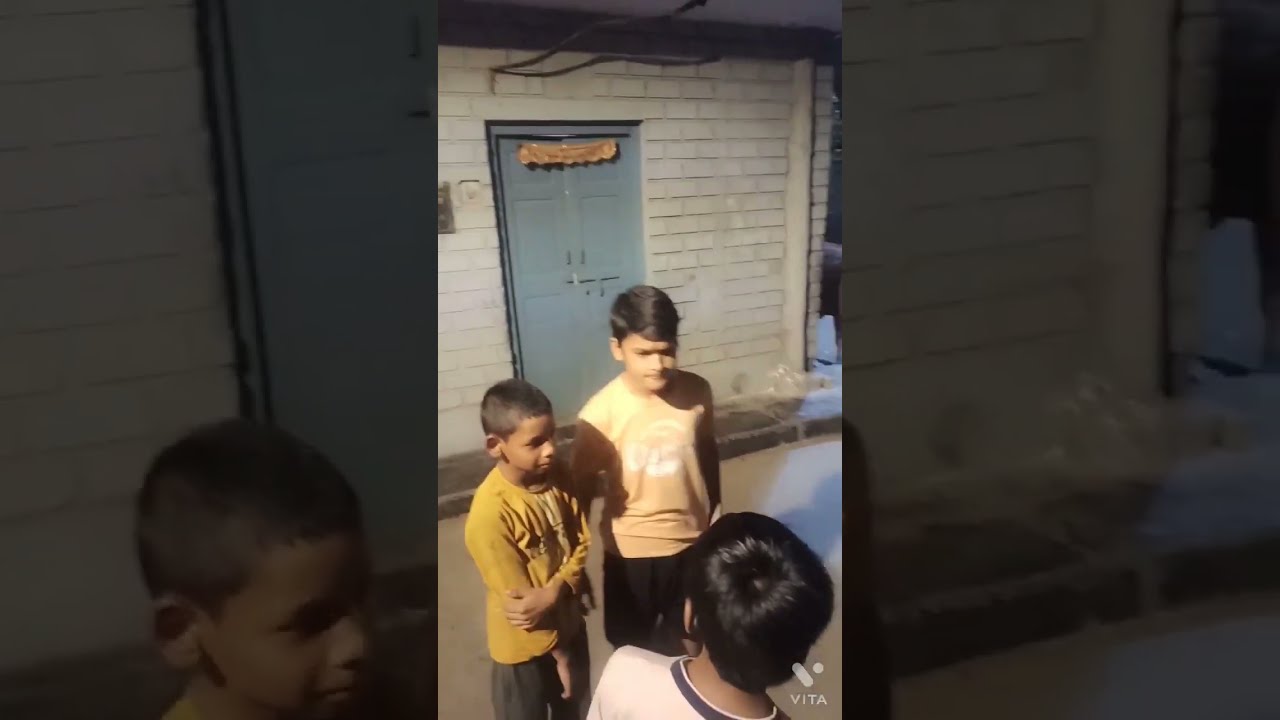The image features three young Asian boys standing in conversation against a gray brick building backdrop, likely either a home or an industrial setup. Central to the composition is a large, light blue rectangular door adorned with an unreadable orange banner. The boy on the left has very short dark hair, wears a long sleeve mustard yellow shirt, and gray shorts or black pants, with one arm casually crossed over his chest. To his right, another boy sports a short sleeve peach-colored shirt with white text on the front and black shorts. Facing away from the camera is a boy with dark black hair and brown skin, dressed in a white t-shirt featuring a black collar. The setting, further suggested by the gray surface they stand on, appears modest with a potential school vibe, and a text reading "VITA" is faintly visible in the lower right-hand corner of the image.